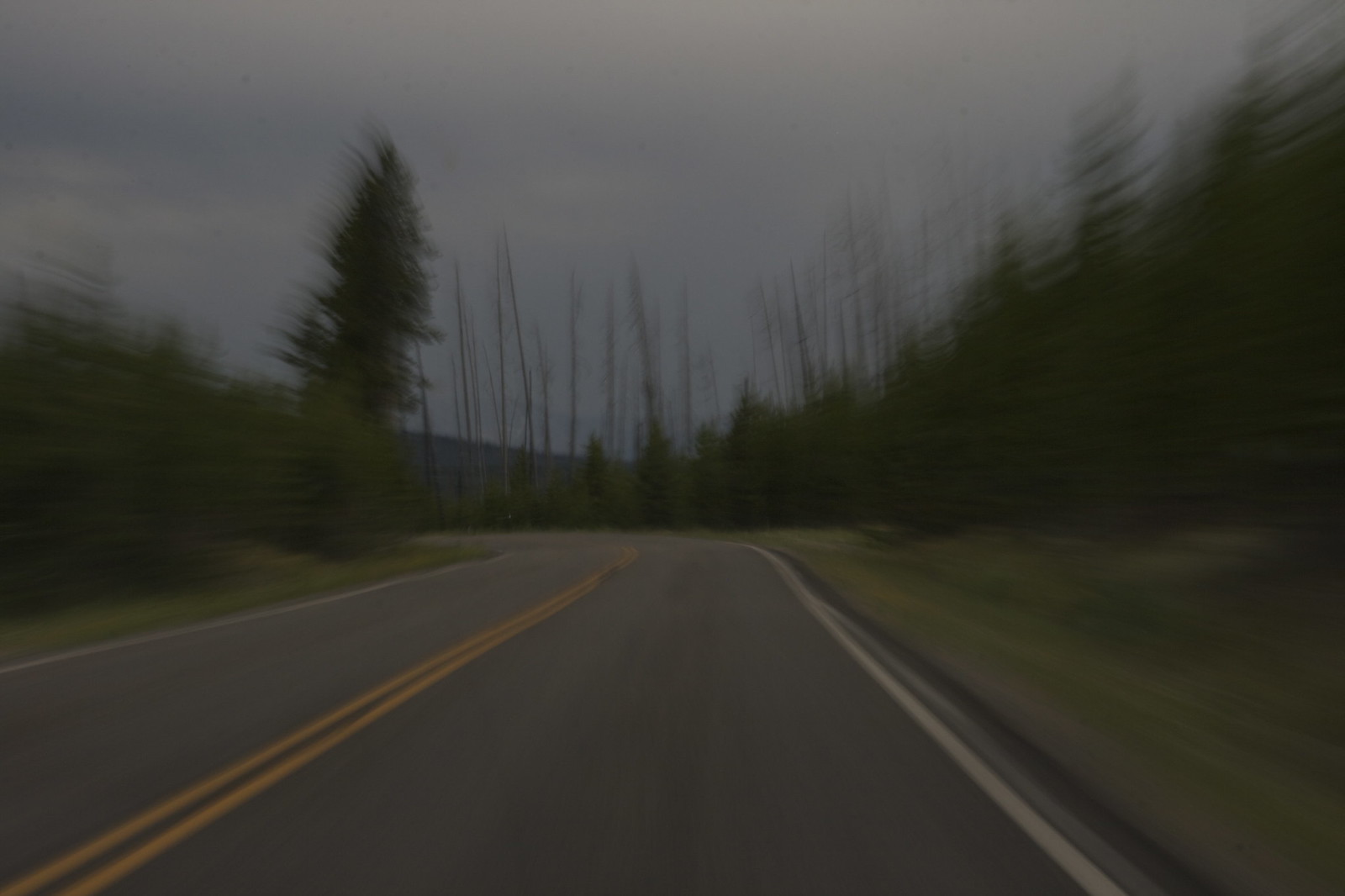The photograph depicts an evening scene taken from the perspective of a moving vehicle, likely through the windshield, making the image slightly out of focus and dark, hinting at either dusk or early morning. The road, an asphalt-paved two-lane highway, features a double yellow line down the center and white lines along the edges. It curves to the left in the horizontal frame, starting in the lower left and extending forward. On the right side of the road, there's a curb, while both sides are bordered by grassy areas leading up to a mix of tall fir-like trees and barren trees lacking foliage. The sky above is heavily clouded, with a blue-gray, foggy, or overcast atmosphere, and faint hints of a horizon with hills in the distance.